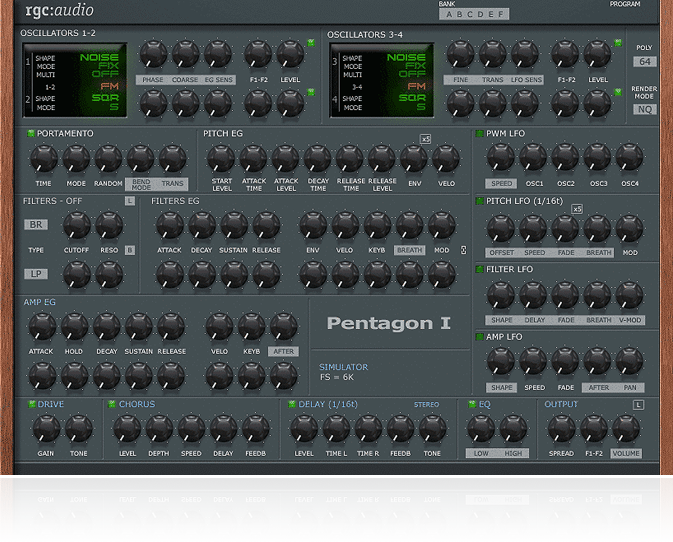This photograph captures a detailed view of a professional music-mixing equipment console, bordered on either side by narrow vertical bands of wood grain. The central area has a dark gray background adorned with numerous black knobs and switches. The top left corner prominently displays the name "RGC Audio" in white text. Further to the right, the labels "Bank ABCDEF" and "Program" are visible. The layout features a series of organized sections: "Oscillators 1-2" next to "Oscillators 3-4," followed by "Portamento," "Pitch," "PWM," "Filters," "Filters EG," "Pitch LFO," "Amp EG," "Amp LFO," and "Simulator FS-6K." An area in the middle is labeled "Pentagon 1." Along the bottom, additional labels include "Drive," "Chorus," "Delay," "EQ," and "Output," completing the intricate array of controls designed for sophisticated audio manipulation.